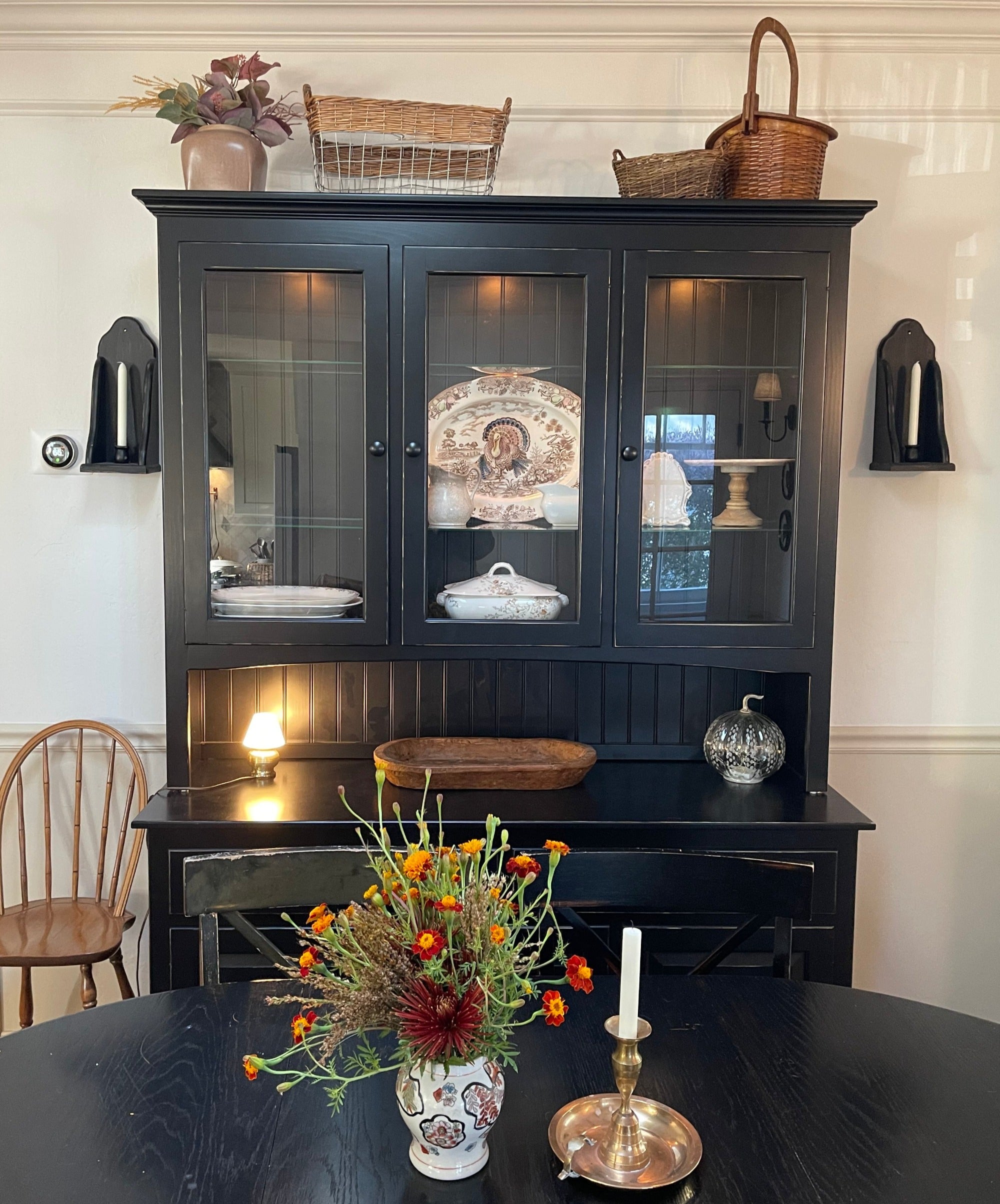This detailed image depicts an elegant dining room, centered around a black wooden hutch or china cabinet, positioned against a light tan wall. The hutch features a base section with multiple drawers, topped by a smooth surface holding an array of decorative items: a wooden oval bowl, an electric lamp on the left, and a silver globe-like ornament on the right.

Above this, the hutch has three clear glass doors, revealing shelves adorned with fine china. The left shelf holds oval white dishes, while the middle shelf showcases a white casserole dish with a lid, a white oval plate with intricate red, gold, and yellow designs standing upright, and a large turkey platter. The right shelf includes a brown cake pedestal and various ornate items.

Flanking the hutch on the wall are two black candle holders, each fastened with a white candle. Atop the hutch, additional decor includes a brass flower pot with brown and green leaves on the left, a wire basket, and two brown baskets to the right – one woven with a handle and the other rectangular with small end handles.

In front of the hutch stands a round black wooden table with a metal dish on the right, holding a gold candlestick and white candle. To the left of this is a white flower pot with colorful designs in black, red, gold, and yellow, filled with green-stemmed red and yellow flowers. Two black wooden chairs accompany the table. On the floor to the left of the hutch sits a wooden chair with a flat seat and a curved back, supported by five vertical sticks. This harmonious arrangement creates a balanced and inviting dining space.